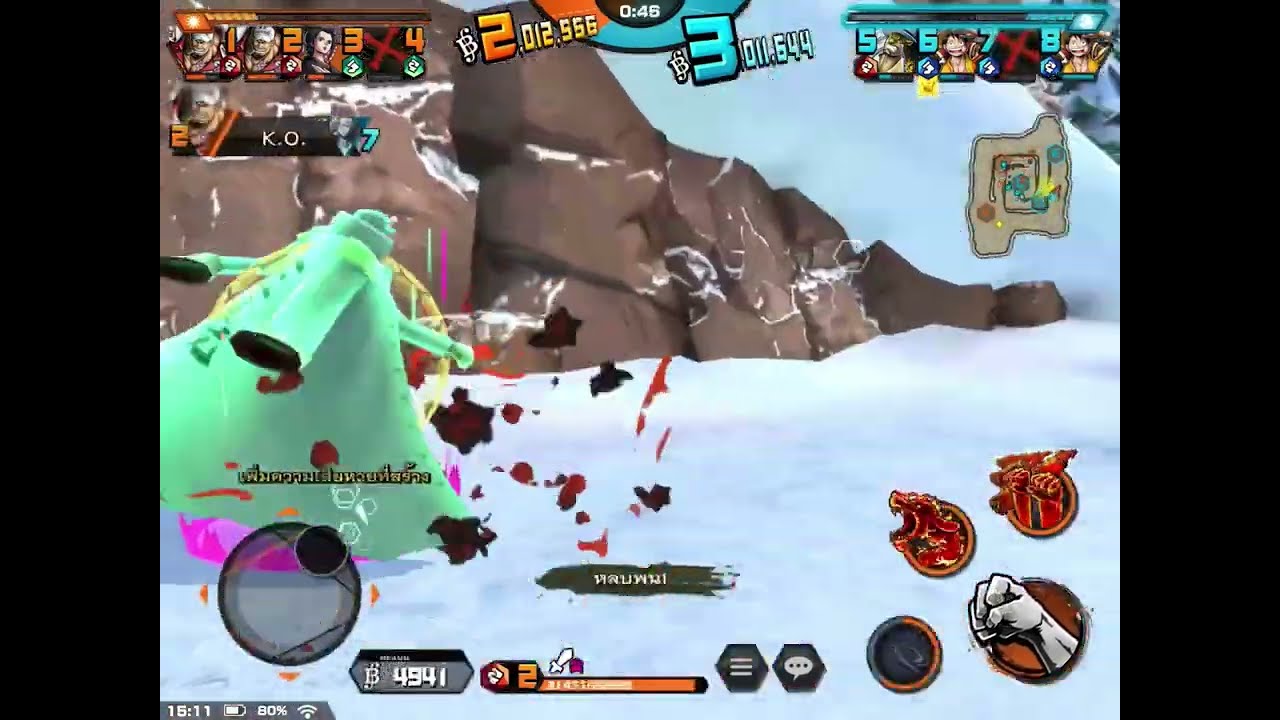The screenshot captures an intricate interface from a computer game set in a snowy, rocky terrain. On the left side, a giant creature or human figure wearing a green robe, detailed with some pink and black elements, moves rightward. The ground is covered in a thick layer of white snow, and a rugged mountain with large rocks forms the backdrop. The game interface features thick black borders on both sides.

The top left corner of the screen displays character icons numbered 1, 2, 3, and 4, while the top middle features an array of numbers such as "0:46," and others like "2.0," "2.5," "5," "6," "3.0," "1.6," and "4.4." In the top right corner is a small brown maze, accompanied by more character icons numbered 5, 6, 7, and 8, underneath which a small map offers a glimpse of the game world. 

A detailed array of stats is visible throughout the interface, including points totaling 4941 highlighted in a gray tab at the bottom, a central timer set at "0:45," and various other numeric indicators. Icons such as a lion in a bubble, another object in a bubble, and a white fist in a bubble are also present. 

The bottom left corner reveals phone stats, showing the time "15:11" (or 3:11 PM in standard time), an 80% battery level, and a strong Wi-Fi signal. The bottom right corner includes additional icons flanked by circles, enhancing the game's detailed interface.